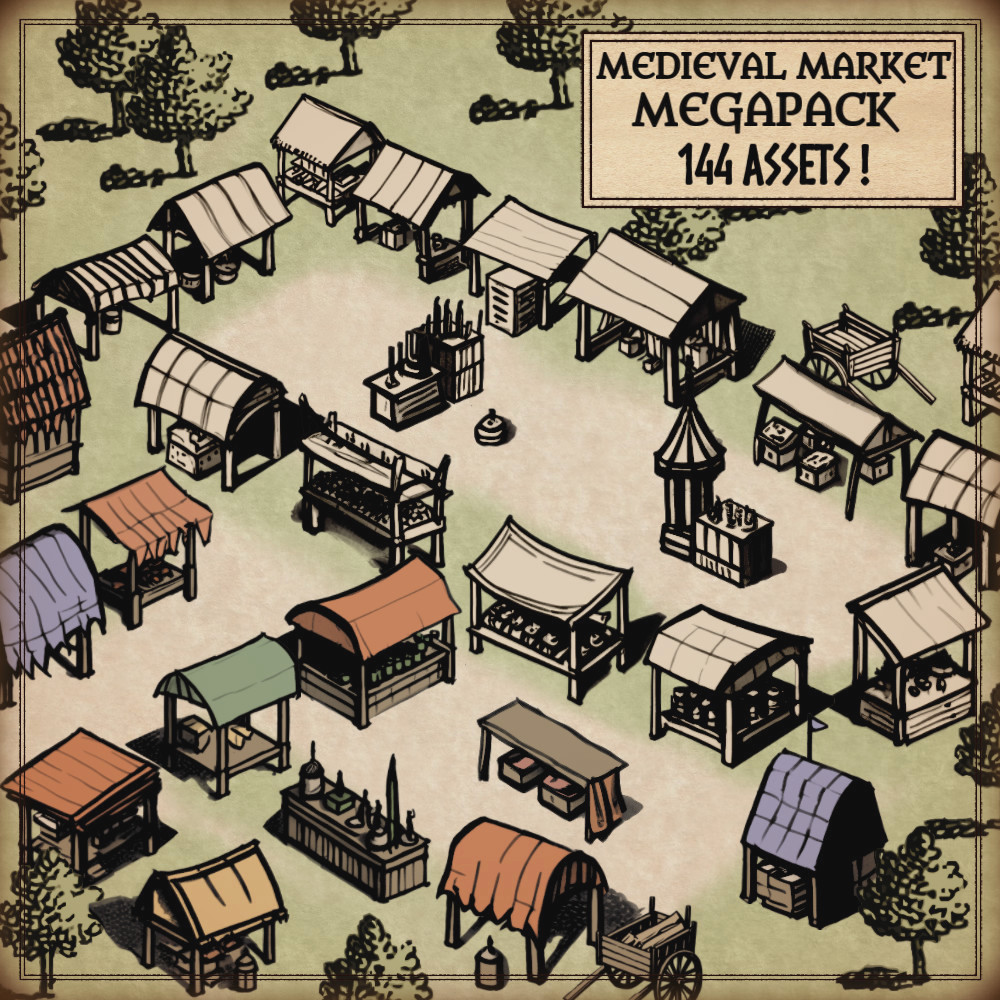This color illustration, set against a light green background, features a detailed square scene bordered by a thin black line. The upper and lower edges of the scene are densely populated with trees, lending a natural feel to the setting. The focal point of the illustration is a collection of various small market huts and wooden carts arranged side by side. These structures, reminiscent of a medieval marketplace, boast roofs in several colors, including white, orange, green, light purple, red, and blue. The materials and styles give the sense of a bustling, vibrant market, though no people are depicted.

A light beige, horizontally rectangular plaque is positioned in the upper right corner of the illustration. It contains black text in an ancient font that reads "Medieval Market Mega Pack 144 assets!" This text block adds context to the scene, suggesting that the image is promotional material for a cartographic accessory pack. The dense array of differently colored roofs and rustic market elements, along with the surrounding trees, creates an intriguing and engaging visual representation of a medieval market.